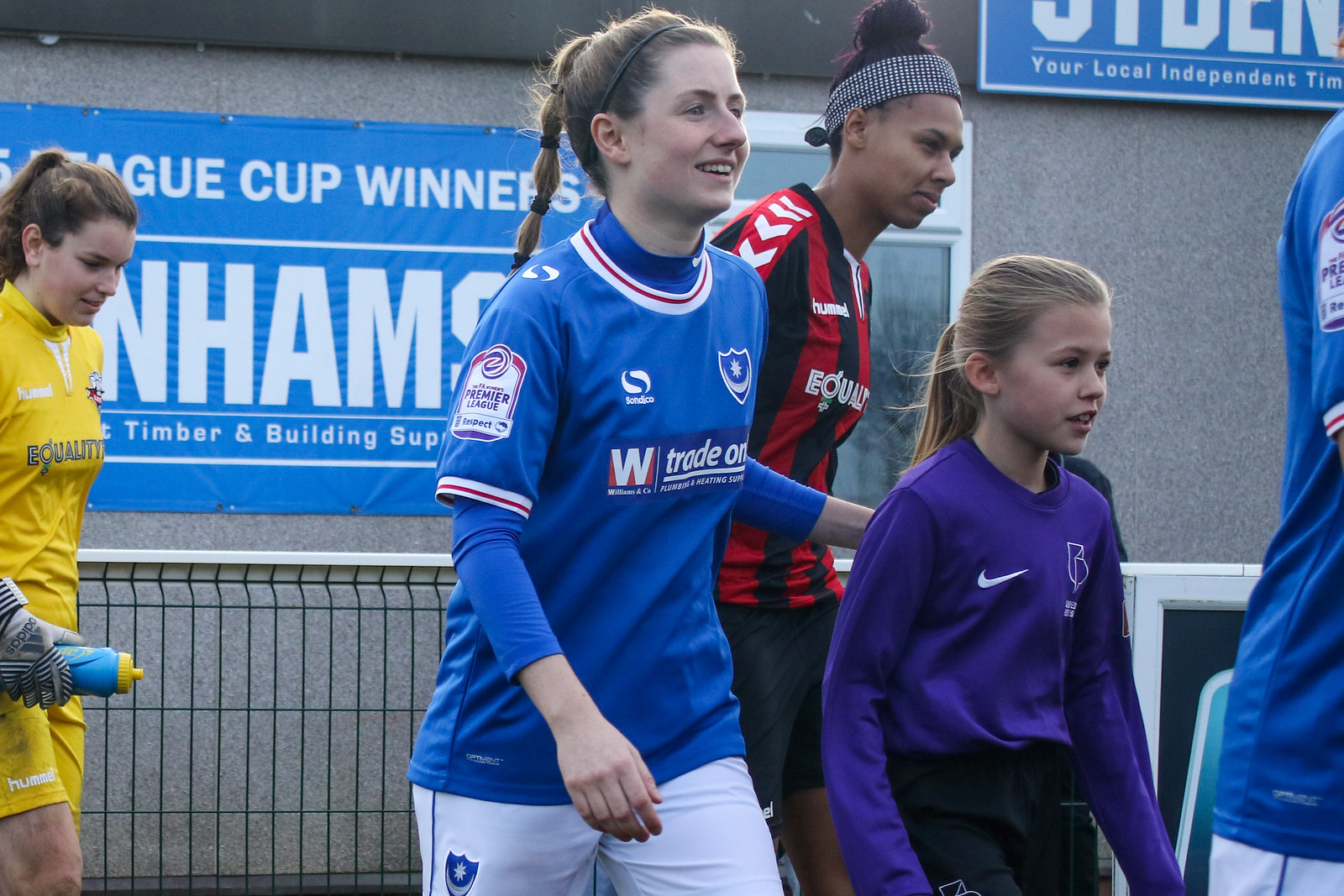In this photograph taken outdoors, five individuals are gathered in front of a gray brick wall with a partially obscured banner that reads "League Cup Winners" and mentions "Timber and Building Supplies" as a possible sponsor. The central focus is on a group of young women who appear to be part of a soccer team. 

On the far left, a teenage girl in a yellow soccer outfit, complete with yellow top, shorts, and gray gloves, is looking down at a blue water bottle with a yellow cap. Next to her, a teenage girl stands out in a blue soccer jersey adorned with various patches and a prominent "W" along with the words "trade one." She has a ponytail and places her left hand gently on the back of a young girl in a long-sleeved purple top with a Nike swoosh, who appears to be about 10 years old. 

Behind these two young girls is a taller woman of African descent, sporting a red and black vertically striped jersey with some writing that reads "E-D-U-I-Z." Further right, we get a glimpse of another figure wearing a similar blue top as the central girl, their back turned towards the camera. The backdrop includes gray bricks and another partially visible blue sign with white lettering that seemingly repeats the information on the main banner. The overall scene is bright, suggesting it is midday, and captures a moment of camaraderie among the soccer players.